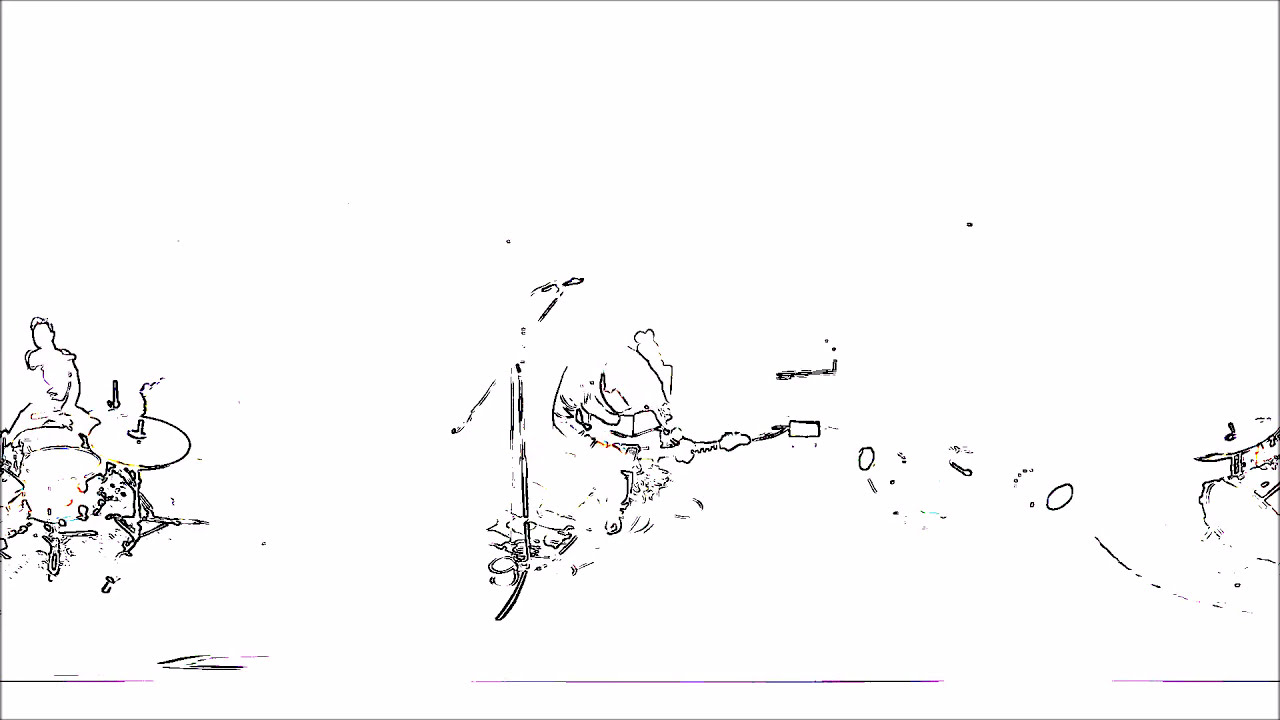This image is a sketch drawing, formatted in a horizontal rectangular shape, with a white background and a thin black line outlining the rectangle. The drawing appears to be black and white, possibly created by a computer. Spanning from just below the center and stretching from left to right, the image showcases several distinct sections of scribbled lines and shapes.

On the far left, there's a discernible figure, likely a musician, sitting at a drum set, identifiable by the cymbal on a hoist and the drums positioned in front of the figure. Moving towards the center, the scribbles become denser, with a mix of vertical and parenthesis-like lines forming indistinct shapes, some attempting to resolve into squares. The middle section, though somewhat abstract, suggests the presence of a wall or piece of machinery, contributing to the overall theme of a musical setup.

Advancing to the right, you'll spot several small circles and another drum set, this time without any figure playing it. The drawing includes the silhouettes of musicians and the outlines of their instruments, indicating a three-piece rock band complete with drums, a guitar, and a microphone stand. Below the scattered scribble sections, a thin black line runs across horizontally, selectively underlining only where the scribbles are present, with noticeable gaps aligned with the spaces between the scribbled segments.

Despite its incomplete and sketch-like nature, the artwork vividly captures the essence of a rock band, offering a potential album cover if color and titles were added. The artistry lies in its rough yet evocative portrayal of a live musical ensemble.